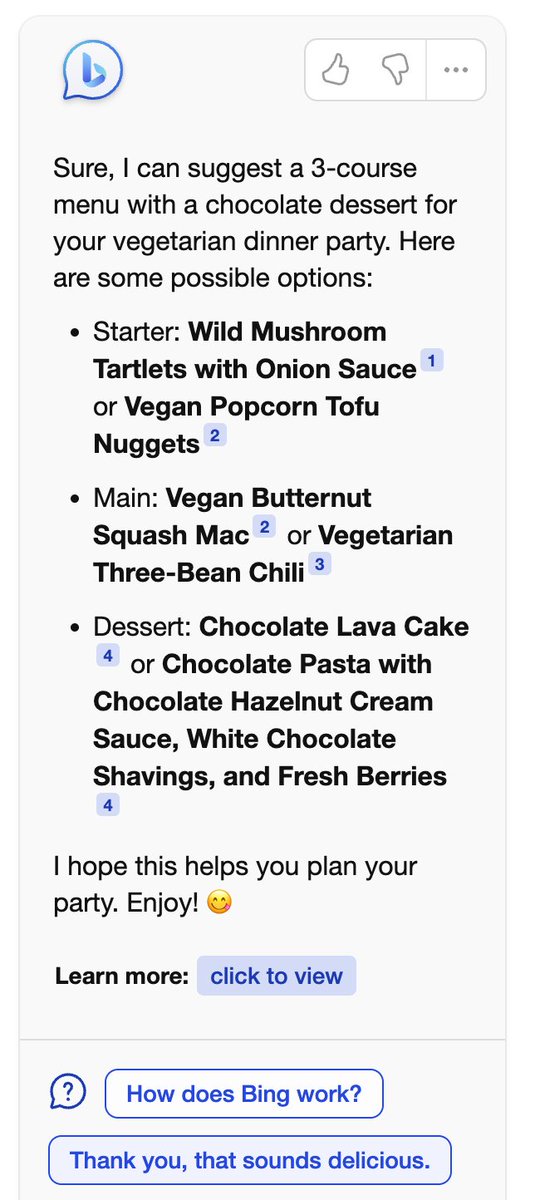Screenshot of a Chat Interface Detailing a Customized Vegetarian Dinner Party Menu:

The screenshot captures a chat interface, presumably powered by Bing. At the top of the screen, the Bing logo is prominently displayed in blue. On the right side, there are icons for thumbs-up, thumbs-down, and an ellipsis for additional menu options.

The chat content, centered against a gray background, showcases a helpful response suggesting a three-course menu with chocolate dessert options for a vegetarian dinner party. The message reads: 

"Sure, I can suggest a three-course menu with a chocolate dessert for your vegetarian dinner party. Here are some possible options:

1. **Starter**: 
   - Wild Mushroom Tartlets with Onion Sauce 
   - Vegan Popcorn Tofu Nuggets

2. **Main**: 
   - Vegan Butternut Squash Mac 
   - Vegetarian Three-Bean Chili

3. **Dessert**: 
   - Chocolate Lava Cake 
   - Chocolate Pasta with Chocolate Hazelnut Cream Sauce, White Chocolate Shavings, and Fresh Berries

I hope this helps you plan your party! Enjoy 😊"

Below the message, there's an option to learn more, indicated by "Click to view." A gray line separates this area from the rest of the interface, followed by a question mark icon. Near the bottom, there are buttons labeled "How does Bing work?" and "Thank you. That sounds delicious." Users can reply back using these interactive buttons. 

Each menu item is numbered (1, 2, 3, 4...), likely linking to detailed recipes or additional information.